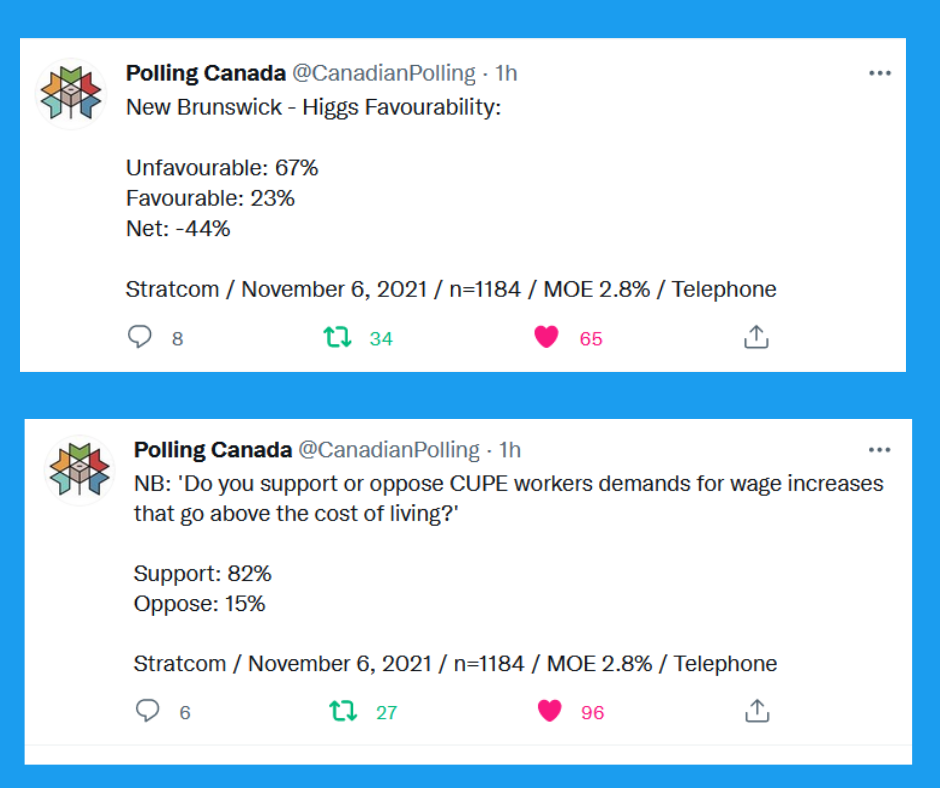This image is a screenshot likely captured from a social media app, though the exact platform is unidentified. The screenshot features two distinct sections, each enclosed in rectangular blue-bordered boxes, positioned one on top of the other against a white background with black text.

The top section displays a small, indistinct insignia resembling a peacock and is labeled "Polling Canada" in bold. Below it reads, "@CanadianPolling - 1 hour ago," indicating the timestamp. The post details a favorability poll for New Brunswick's Higgs, with results showing 67% unfavorable, 23% favorable, and a net favorability of -44%. The poll, conducted by STRATCOM on November 6, 2021, surveyed 1,184 people (N) with a margin of error (MOE) of 2.8%. There are indicators of user interaction: 8 comments, 34 shares (represented by a box with arrows icon), and 65 likes (indicated by a heart icon).

The bottom section, also from "Polling Canada" (@CanadianPolling - 1 hour ago), examines public opinion on the demands of CUPE workers for wage increases above the cost of living. It reveals that 82% support and 15% oppose the demands. This poll was similarly conducted on November 6, with the same sample size of 1,184 (N) and an MOE of 2.8%. User engagement shows 6 comments, 27 shares, and 96 likes.

The image concludes with a note directing viewers to more UN videos at www.un.org.